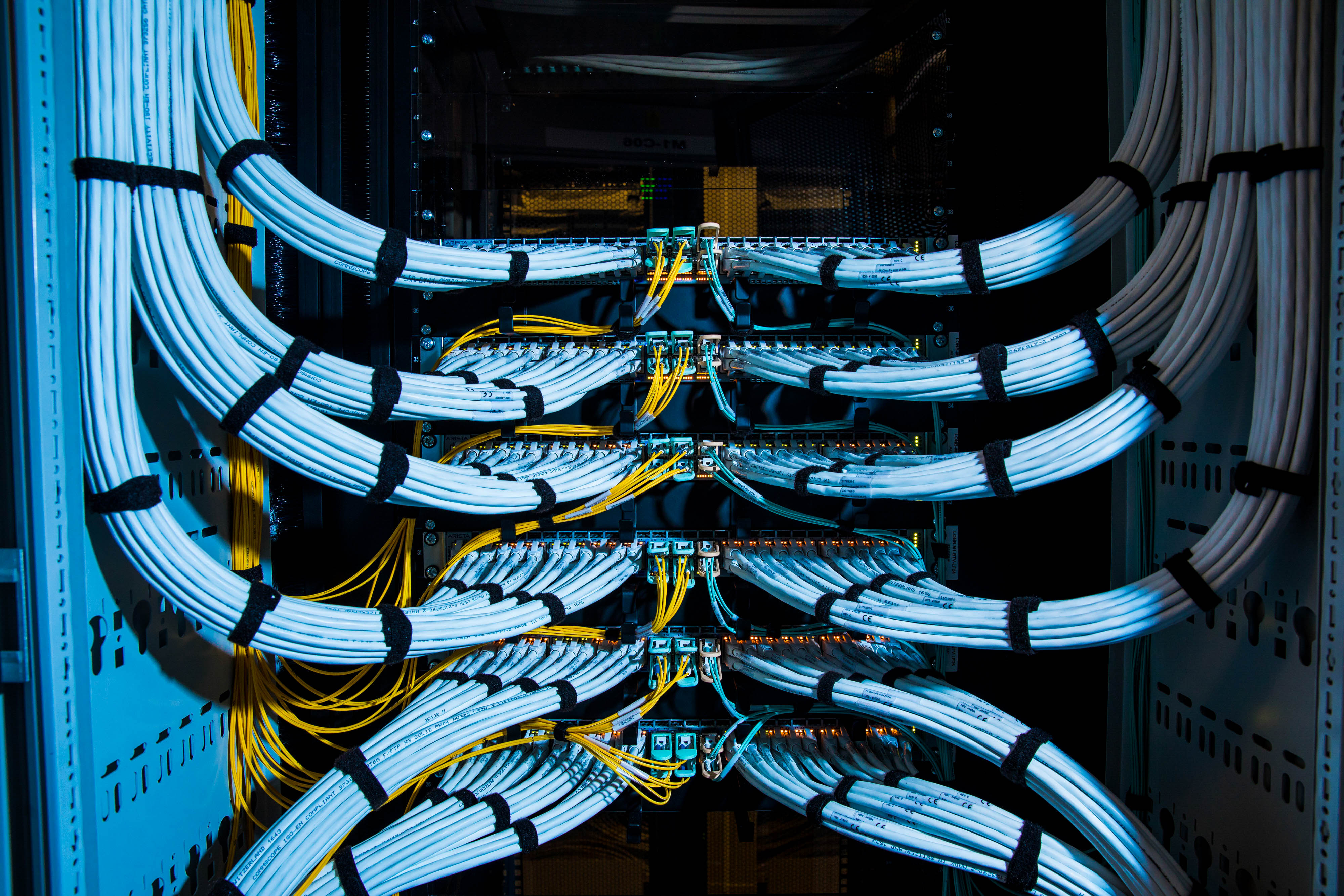The photograph captures the meticulously organized interior of a server rack cabinet. At the center of the image, several server stacks and at least six distinct switch panels are prominently featured. The cabling is impressively managed, with a plethora of cables running both from the top and bottom, curling towards the center where the servers are nested. Two main types of cables dominate the scene: thick white cables, bundled together with black straps, and skinnier yellow cables, also secured by black straps. The image showcases a highly efficient setup with symmetrical clusters of cables on both the left and right sides of each server rack. These are likely Ethernet or Cat5 cables, and they include yellow cables on the left side and some teal or turquoise cables on the center-right of each rack. The cables almost resemble tentacles emanating from the switch panels, contributing to the overall sense of order and clarity in the setup. The interior of the server rack is dimly lit, primarily illuminated by the ambient glow of the cables themselves.